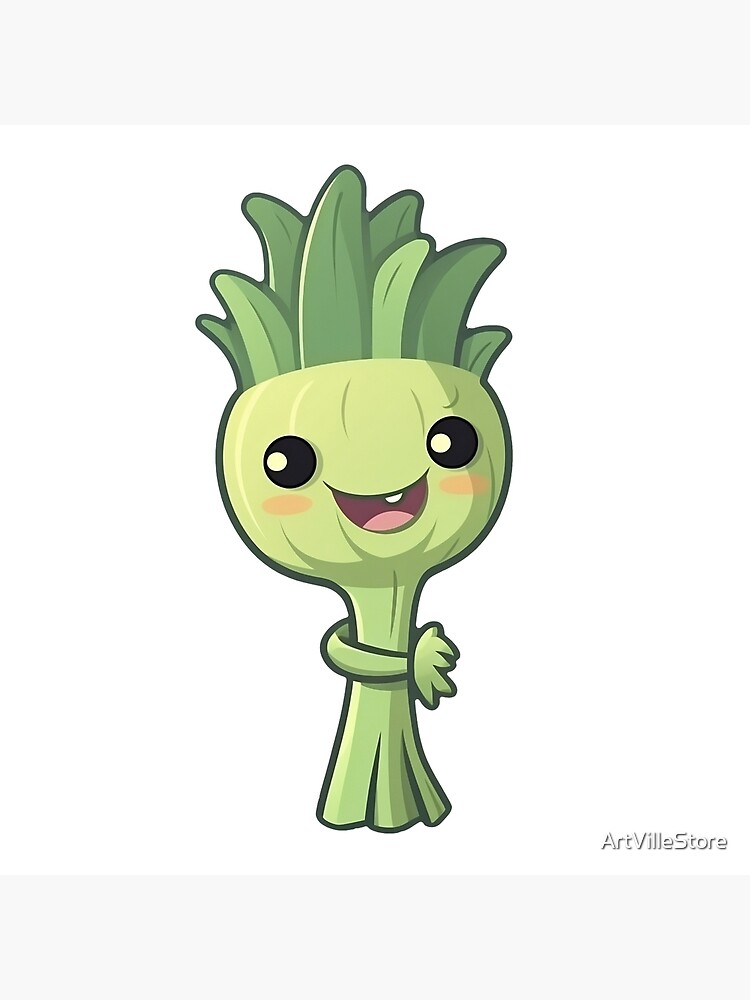The image is a delightful cartoon illustration of a vegetable character set against a white background with a soft grey rectangle at the bottom, which features the text "Art Villa Store" in grey. The character, likely a green onion but ambiguously designed to appear like various types of vegetables, has a round bulbous head with a thin, stalk-like body reminiscent of celery. It has an expressive face, with large black eyes that have white centers, a smiling open mouth showcasing a tongue and a single tooth. The character's cheeks are adorned with peach-colored smudges, hinting at rosy cheeks. At the top of its head, several green, leaf-like structures of varying shades and lengths give the appearance of tufted hair. This charming animated figure is light green in color, with small hands extending from its body, and brings a lively, joyful presence to the image.